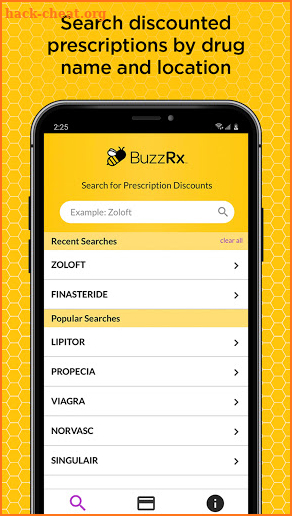This image is a detailed screenshot of an advertisement aimed at promoting prescription discounts. The background features an intricate honeycomb design in an orangey-yellow hue with a crisp white honeycomb pattern overlay. In the top left corner, there's a watermark displaying "hack-cheat.org." Below this, in bold black font, the text reads, "Search discounted prescriptions by drug name and location."

Central to the image is a graphic of a smartphone with a black bezel, displaying a webpage. At the top of the webpage, there's an orangey-yellow rectangle with a bee icon accompanied by the text "BuzzRx." Beneath this header, the text instructs users to "Search for prescription discounts." A gray search field is provided, with placeholder text in gray font that reads, "example: Zoloft," and a small gray magnifying glass icon hinting at its search functionality.

Further down, the webpage has a lighter yellowy-orange section labeled "Recent searches" on the left, with a "Clear all" option to the right in blue font, designed to be clickable. Below this section, there are numerous recent searches listed, each enclosed in a white rectangle. The layout and visual elements are clean and focused on ease of use, promoting quick access to prescription discount information.